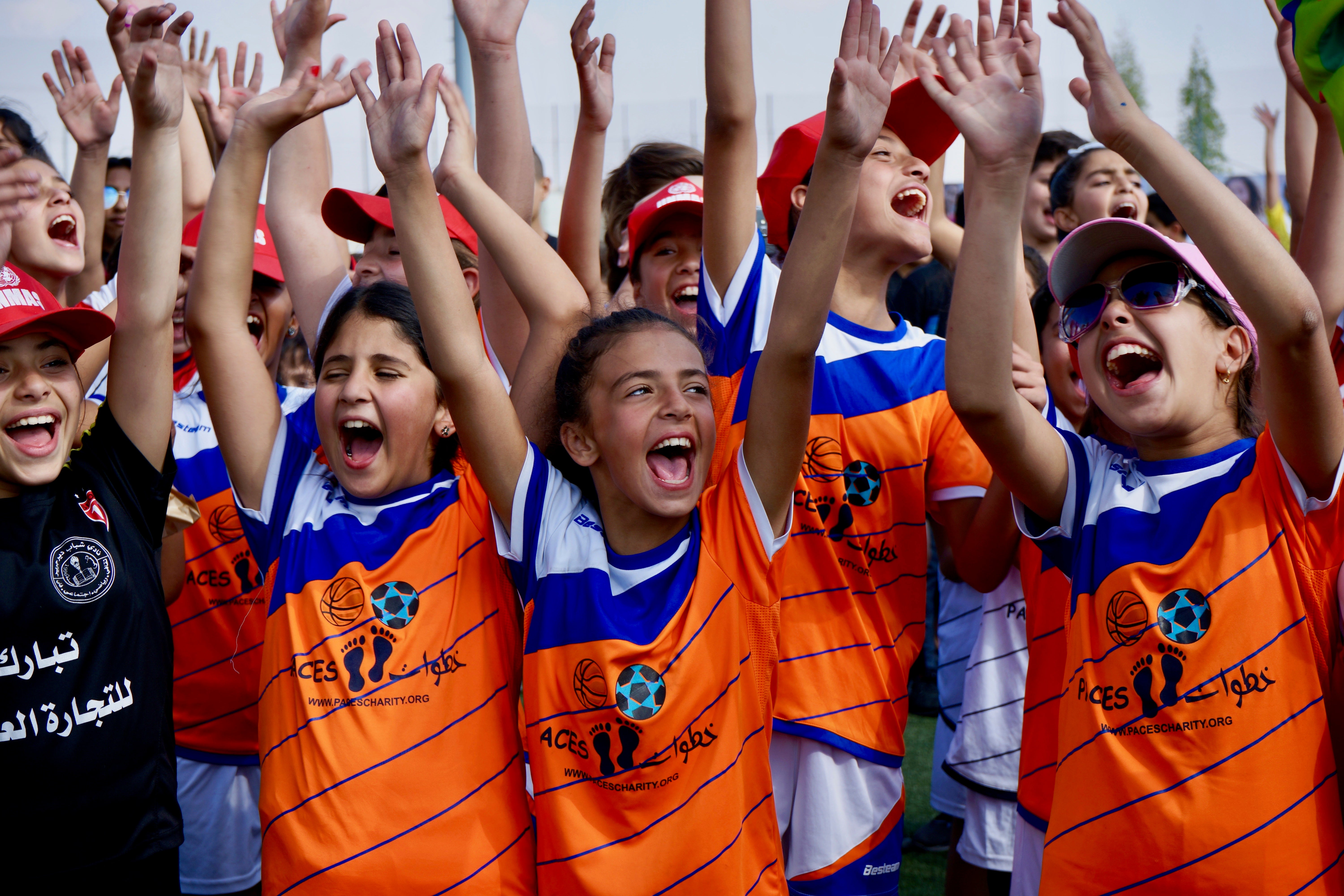The image captures a joyful moment of a group of children in an Arabic country, evident from the Arabic text on their clothing. They are enthusiastically raising their arms in the air, smiling, and cheering. The children are dressed in vibrant jerseys that are predominantly orange, with blue accents such as a crew neck collar, diagonal stripes, and a section near the sleeves. The shirts feature a charitable foundation's logo depicting two footprints, with accompanying images of a basketball and a soccer ball in a cartoon style within the orange section. Some of the children are also wearing visors or hats, with one child on the far right sporting sunglasses. A girl on the left stands out in an all-black shirt and a red baseball cap with Arabic text. The backdrop suggests an outdoor setting where they appear to be engaged in athletic activities or sports games while celebrating their efforts to raise money for charity. The children’s medium complexions and expressive joy create a heartwarming and energetic scene.